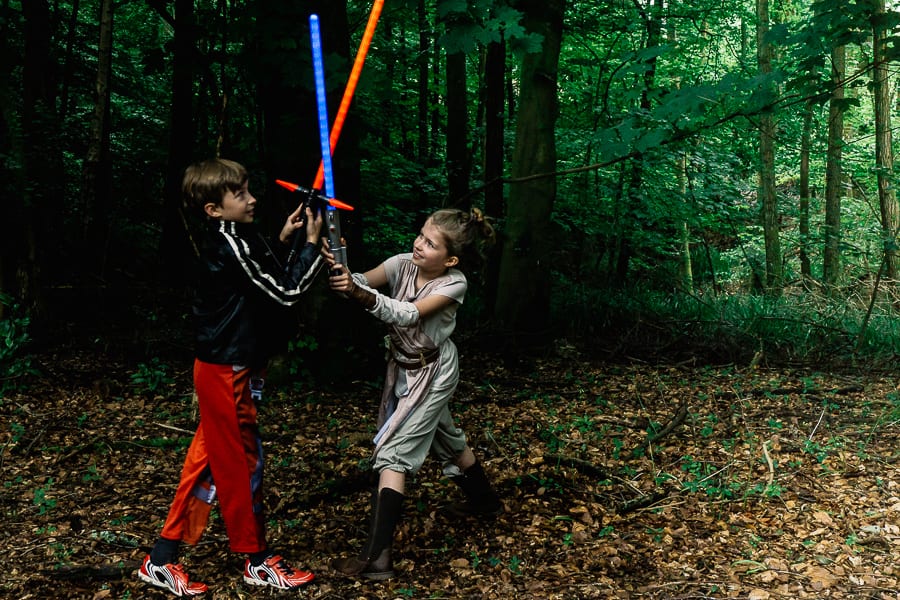In this captivating photograph, two children are immersed in playful combat with plastic swords in a dense forest setting. The little girl, with her hair neatly tied in a ponytail, wields a vibrant blue sword. She is dressed in a t-shirt, long white pants rolled up at the cuffs, and sturdy black boots, reminiscent of a martial arts or superhero outfit. The energetic little boy, sporting short brown hair, brandishes an orange sword. He is clad in orange track pants, a black track jacket, and matching orange and white sneakers, bringing a dynamic splash of color to the scene.

The forest floor is densely carpeted with brown, fallen leaves, under a canopy of tall trees allowing only specks of sunlight to flicker through. The children, with their plastic swords, seem to be engrossed in an epic medieval or fantasy battle, their laughter and spirited movements capturing the joy of imaginative play. Surrounded by a mix of greenery and towering trees with very little sunlight filtering through, the scene depicts the children at the edge of a tranquil, shaded woodland, thoroughly enjoying their adventurous duel amidst nature's serenity.